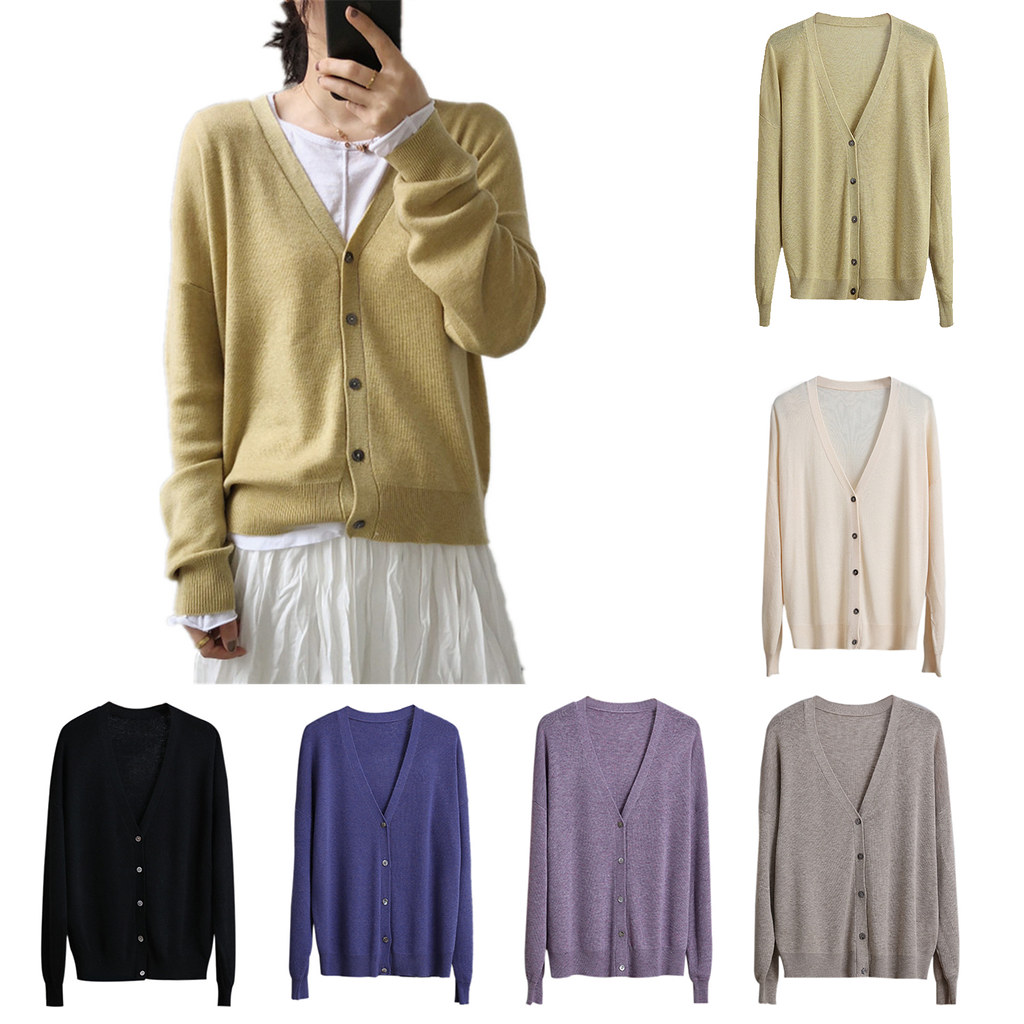The image features a fashion advertisement for a button-up cardigan sweater, taller than it is wide, with a woman modeling the garment from nose to mid-thigh against an indistinct white background. The model, who has dark brown hair pulled back, is wearing a white long-sleeve blouse underneath the light tan cardigan and a matching white skirt. The cardigan, characterized by five buttons and a V-neck, is slightly more tan than mustard in color. The model's face is obscured as she holds a phone in front of it.

To the right and bottom of the model, forming a backwards L shape, are swatches showcasing the cardigan in various colors. Along the bottom from left to right are black, blue, purple, and gray versions. Vertically along the right side are off-white, the tan the model is wearing, peach, and periwinkle blue. The cardigan’s buttons vary, with the lighter purple, periwinkle, and black versions featuring lighter buttons, such as silver or white, while the others have brownish-black buttons.